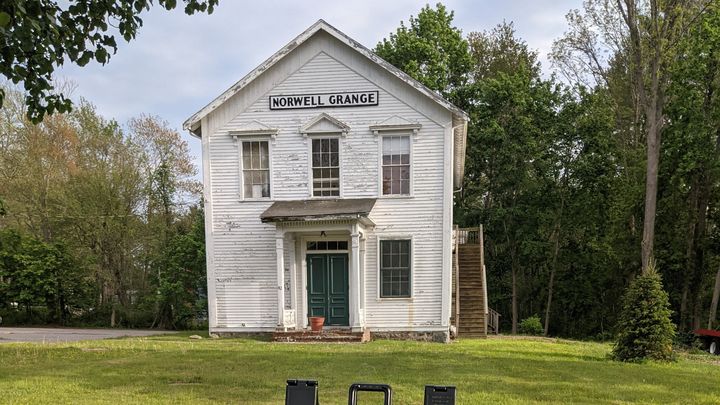In the image, we see the front of a two-story house with a very light gray or white exterior. The house prominently features a green door framed in white, preceded by two brown steps leading up to it. To the right of the door, there is a single gray window. Above, the second level displays three additional windows. At the very top of the house, a rectangular sign reads "Norwell Grange" in black text. A wooden staircase with about 15 steps is visible on the right-hand side of the house. The front yard is covered in grass, and surrounding the house are trees with dark green leaves. The background sky is a clear, light blue.